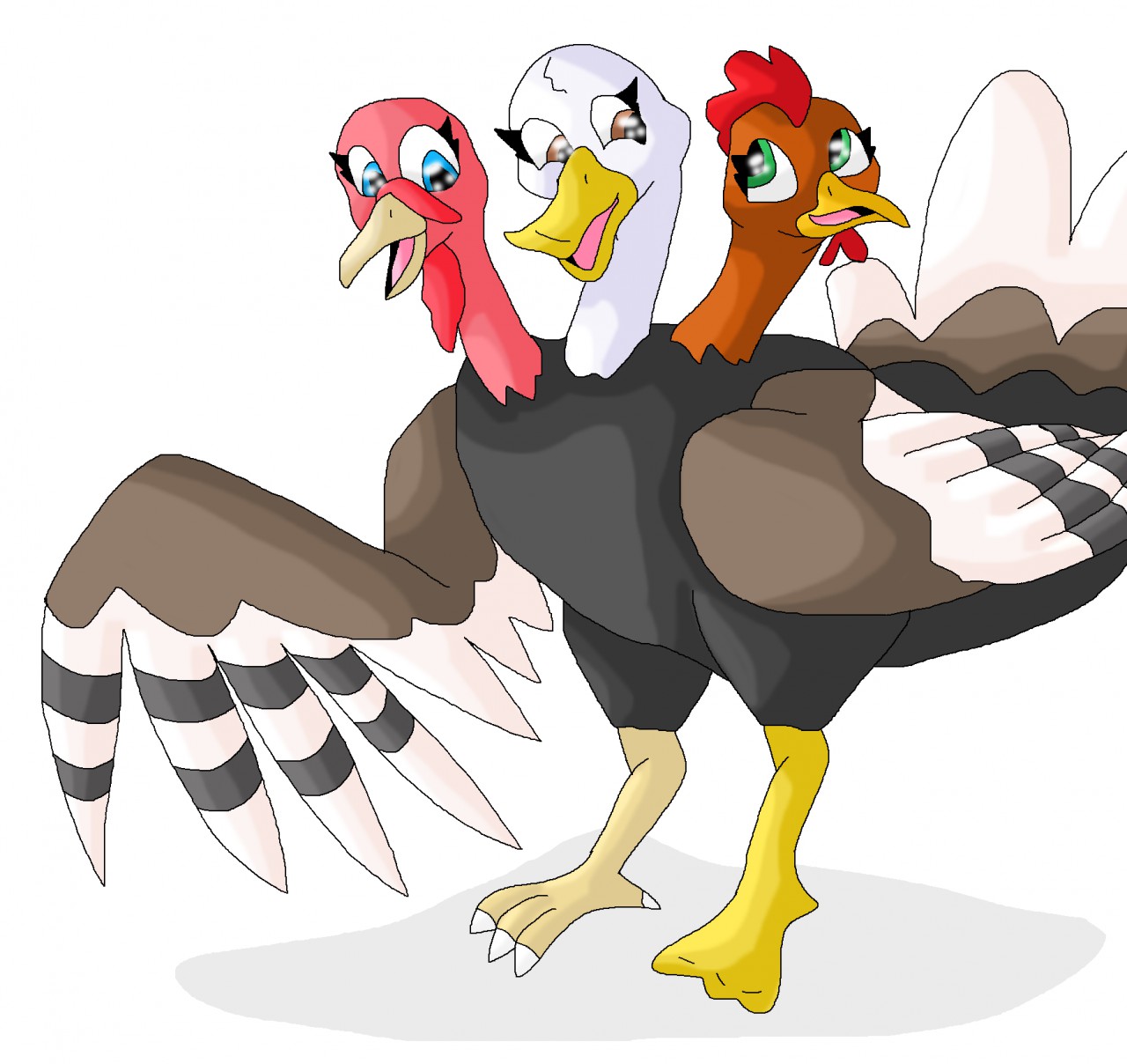This is a cartoon drawing of an unusual three-headed bird-like creature standing on a gray triangular patch against a white background. The body resembles a mix of a turkey and an eagle, primarily black with a dark gray square on the chest highlighting a lighter gray inside. The bird's detailed wings are brown with white tips and distinct black stripes midway. It possesses two distinct legs; the right leg is flesh-colored with white nails akin to a chicken's foot, and the left leg is yellow, resembling a duck's webbed foot. The creature's three heads, from left to right, include: a pink turkey head with a beige beak characteristic of a turkey, a white duck head with a yellow beak, and an orange chicken head with a yellow beak and a tuft of red feathers. The eyes have a stylized, cartoonish quality reminiscent of anime or Disney characters. The entire drawing features proportions that appear somewhat off, giving it an amateurish charm.